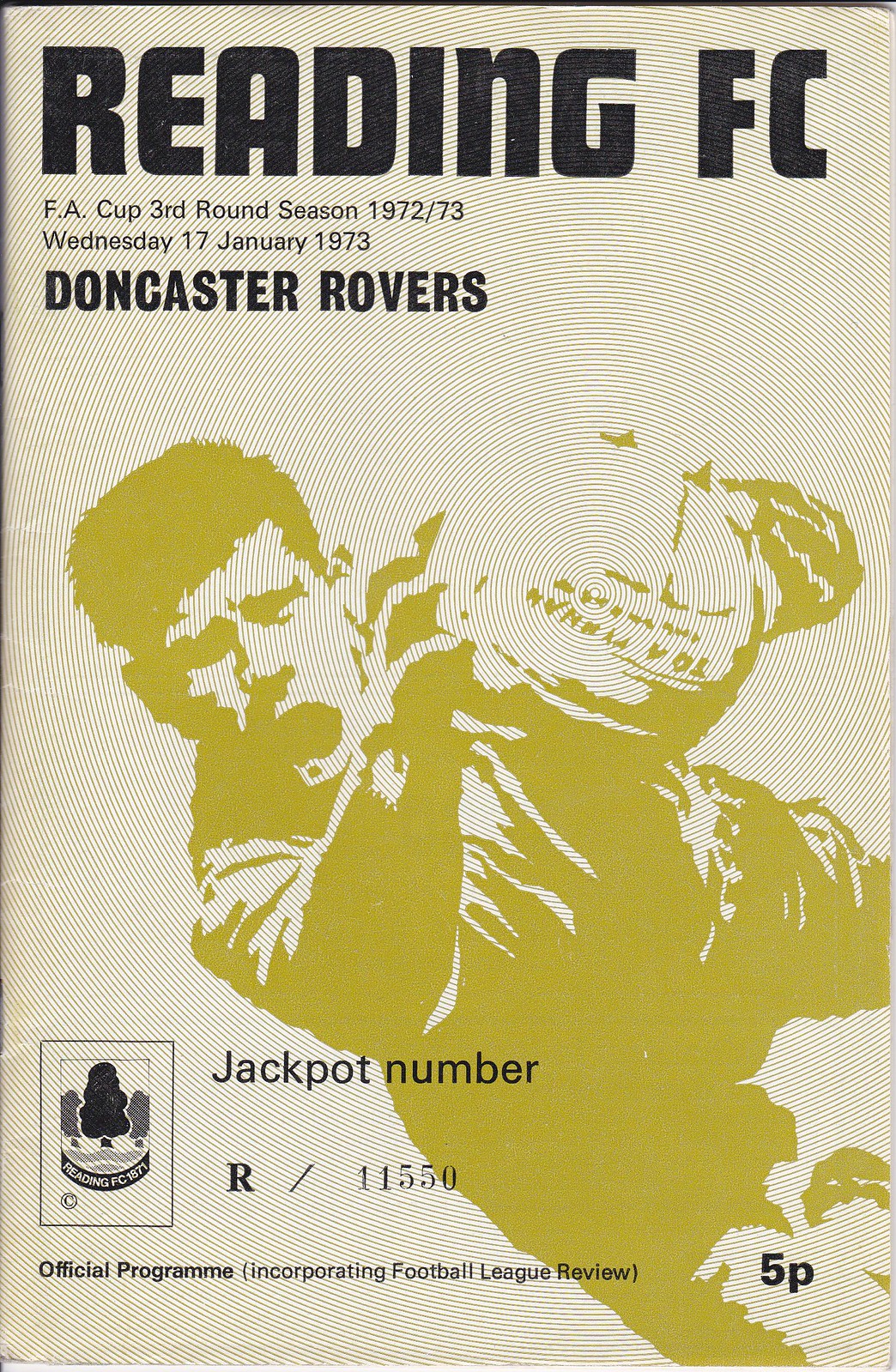This image is an official program for a soccer match with a primarily grayish-green background and bold black lettering at the top. The text prominently reads "Reading FC" followed by "FA Cup, Third Round Season 1972-73, Wednesday, 17 January 1973," and "Doncaster Rovers." A central illustration in brownish-white tones depicts a man, likely a goalie, clutching a soccer ball, characterized by his dark hair and long-sleeved shirt. Below the image, it states "Jackpot Number R/11550." The left side of the program mentions "Official Program, Incorporating Football League Review,” while the bottom right corner lists the price as "5P." There is also a tree-like logo beside the jackpot number, representing Reading FC, though the exact historical year is unclear.